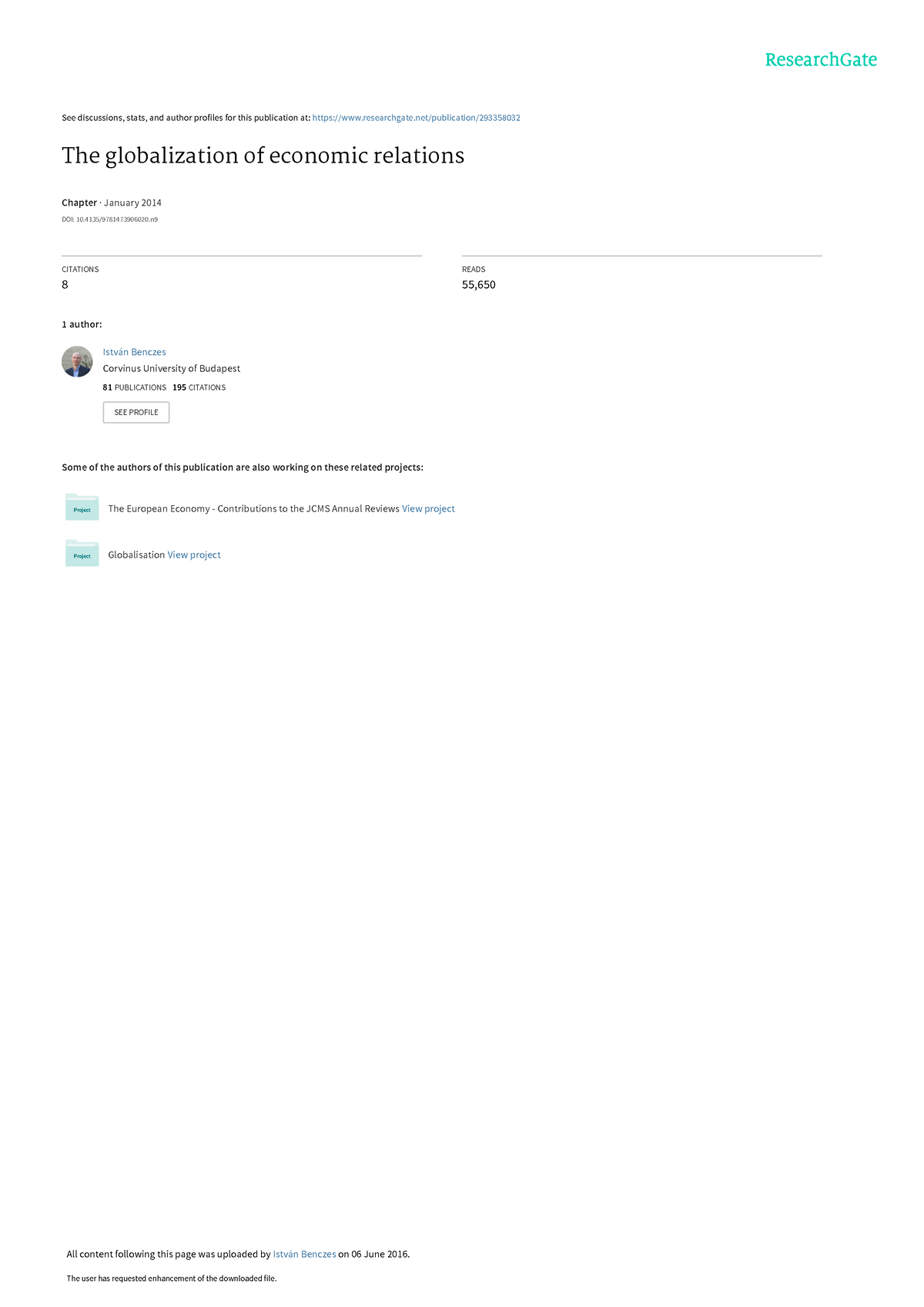Here is a cleaned-up and detailed caption for the described image:

---
Screenshot of a ResearchGate webpage displaying details of a publication titled "The Globalization of Economic Relations." At the top right, the page features the ResearchGate logo in a greenish-teal color. Beneath the logo, on the left-hand side, a small note reads, "See discussions, stats, and author profiles for this publication at," followed by a clickable URL in blue.

The main content starts with the publication title, "The Globalization of Economic Relations," labeled as a chapter with a posted date of January 2014 and an accompanying DOI number. Below the title, statistics are presented in two lines indicating "8 Citations" and "55,650 Reads." 

A circular profile picture appears next, showing a bald man in a dark suit and blue shirt. His name, "Istvan Bankses," is displayed in blue text to the right, along with his affiliation, "Cornelius University of Budapest," where he has 81 publications and 195 citations.

Highlighted in gold below the author information, there is a note indicating that "Some of the authors of this publication are also working on these related projects." Two blue manila folder icons follow, each labeled "Project." The first project is titled "The European Economy: Contributions to the JCMS Annual Reviews," with a "View Project" link beside it. The second project is labeled "Globalization," also featuring a "View Project" link.

At the very bottom of the page, a note states, "All content following this page was uploaded by Istvan Bankses on 06 June 2016." The final line reads, "This user has requested enhancement of the downloaded file."

---
This caption provides a comprehensive overview of the webpage, capturing all the relevant details.